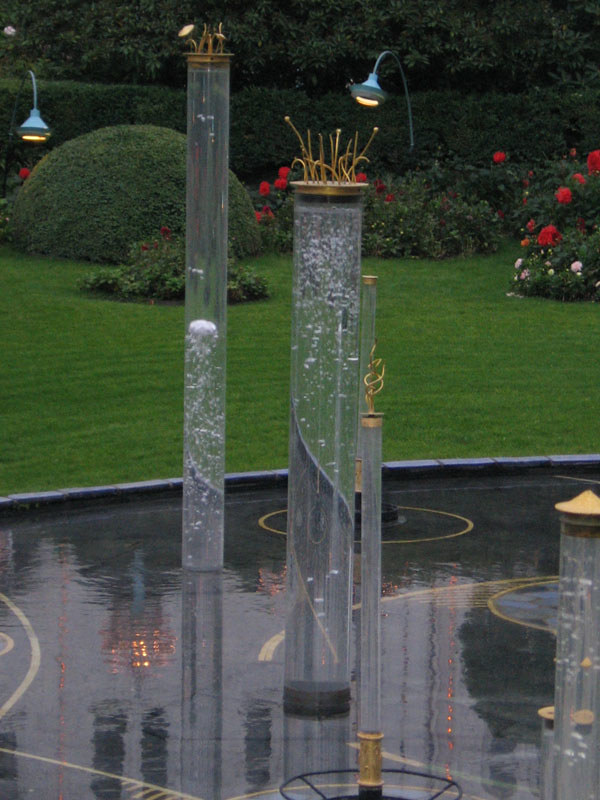The outdoor image depicts a lush garden scene with a variety of greenery and intricate water features. The background showcases dense, dark green trees, bordered by an even hedge that frames the area. Moving forward, the garden features a mix of bushes, including a large round domed bush and several flowering bushes with striking red and pink blooms.

In the foreground, a paved area surrounds a small pool of water from which glass-like cylinders of varying sizes emerge. These cylinders are filled with bubbling water and adorned with gold caps, each featuring delicate gold tubes with small round balls at their tips. Some of the tubes are tall, others shorter, and they create a dynamic visual display.

A halfway-up concrete barrier runs along the water’s edge, adding a structured element to the scene. Off to the sides, blue floor lights with white bulbs curve over the garden, casting a gentle glow. This vibrant outdoor setting combines the tranquility of natural greenery with the elegance of thoughtfully placed water features and lighting.